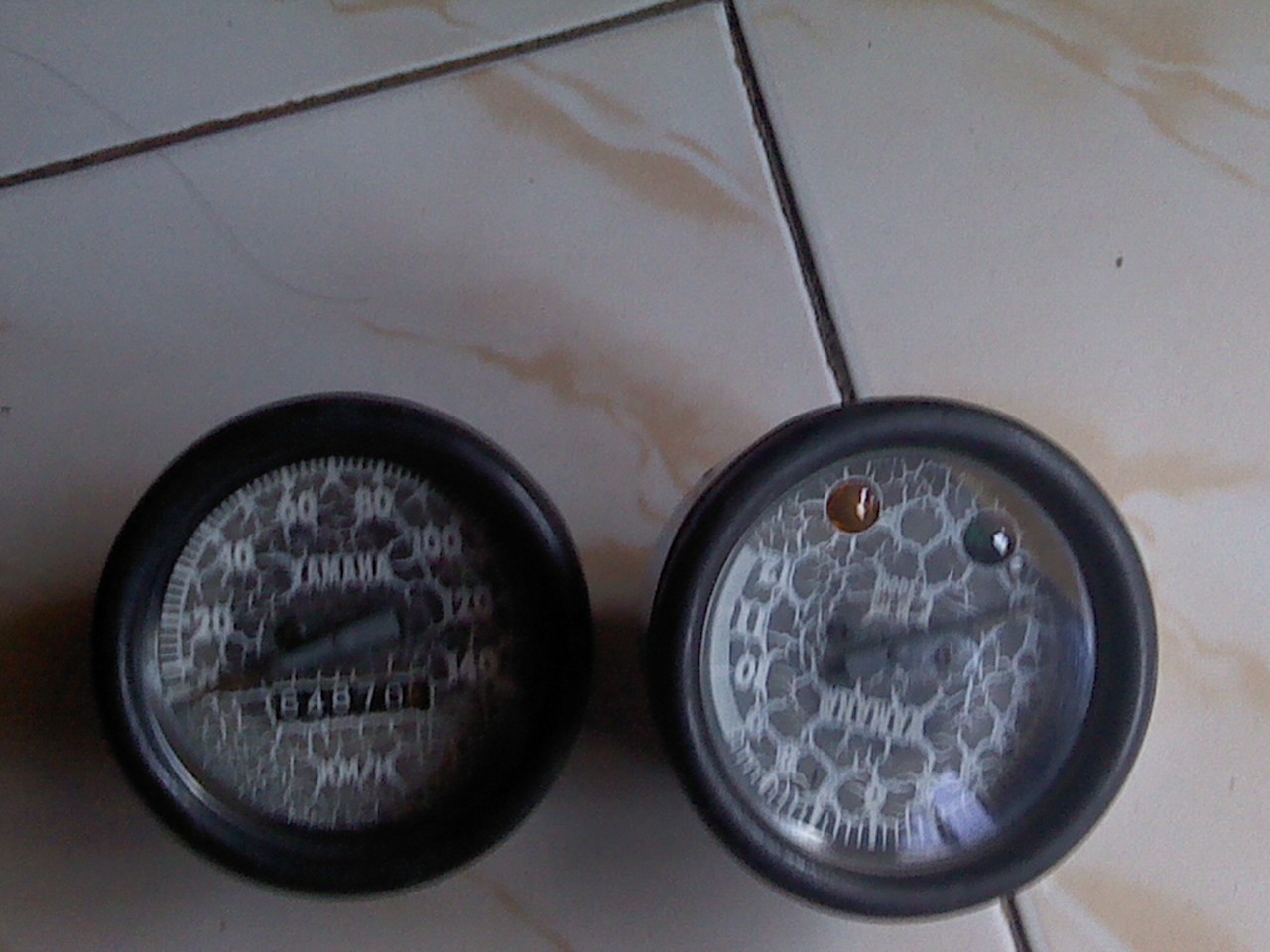The image depicts two disassembled speedometers, likely from a Yamaha motorcycle, placed on a marbled tile floor featuring cream and rust hues. The first speedometer, branded Yamaha, displays an odometer reading of 64,870 miles. Its background is gray, adorned with intricate white crackled lines that obscure some of the finer details, making them hard to decipher. The speedometer's numerical indicators for miles per hour are marked in white, and a black rim encircles the instrument. Beside it, the second speedometer shares a similar color scheme with a black rim. Inside this speedometer, there is an amber light and a green light positioned at the top, both situated above a gray needle that, like the first, moves to indicate speed. A delicate spiderweb-like pattern is present on its face, adding to the intricacy but also contributing to the difficulty in reading the small inscriptions. Both speedometers rest unattached to any vehicle, emphasizing their placement on the patterned tile surface.